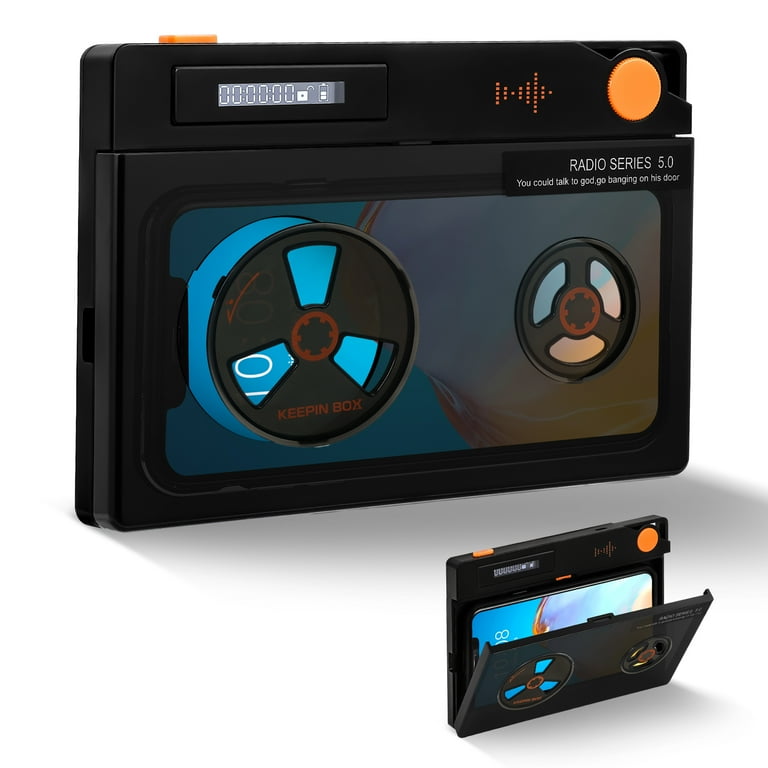The image depicts a black cassette tape deck phone case designed to hold an iPhone, mimicking an old-school cassette player. The case has an orange button on the top right, likely for volume control, and an orange button on the front right side. The central part of the deck features digital elements that suggest a track display and battery level indicator, alongside a lock symbol. The design includes what appears to be the magnetic tape's wheels with a clear cover through which a smartphone inside is visible. The phone case prominently displays the text "Radio Series 5.0" in white on a black background, accompanied by the phrase "you can talk to God, go banging on his door." The image shows both a zoomed-in and an angled view, with the latter revealing the side where the front cover of the cassette deck is open, further confirming the presence of a smartphone inside. This phone case is showcased against a white background, giving it the appearance of a stock photo commonly used in online shopping.